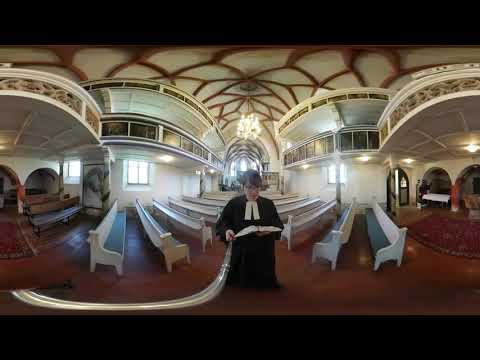The image beautifully captures the serene interior of a church, featuring a kneeling priest or preacher at its center. Clad in flowing black robes and a distinct white collar resembling an inverted V, he is intently reading a holy book. The clergy member wears glasses and is positioned on a brownish-red carpet amidst the church’s ornate ambiance.

Surrounding him are white pews, upholstered with greenish-blue seats, extending from the foreground to the background, where they culminate near an arched window. The church’s walls are also white, contributing to a pristine and tranquil atmosphere. 

The ceiling is an artistic masterpiece with sculptured, flower-like patterns in white and brown, further adorned with red geometric designs that resemble igloos, highlighted by overhead lighting. The space is flanked by arches on either side, hinting at adjacent areas with benches or tables although their exact details remain indistinct. The overall setting exudes a harmonious blend of color, structure, and reverence.